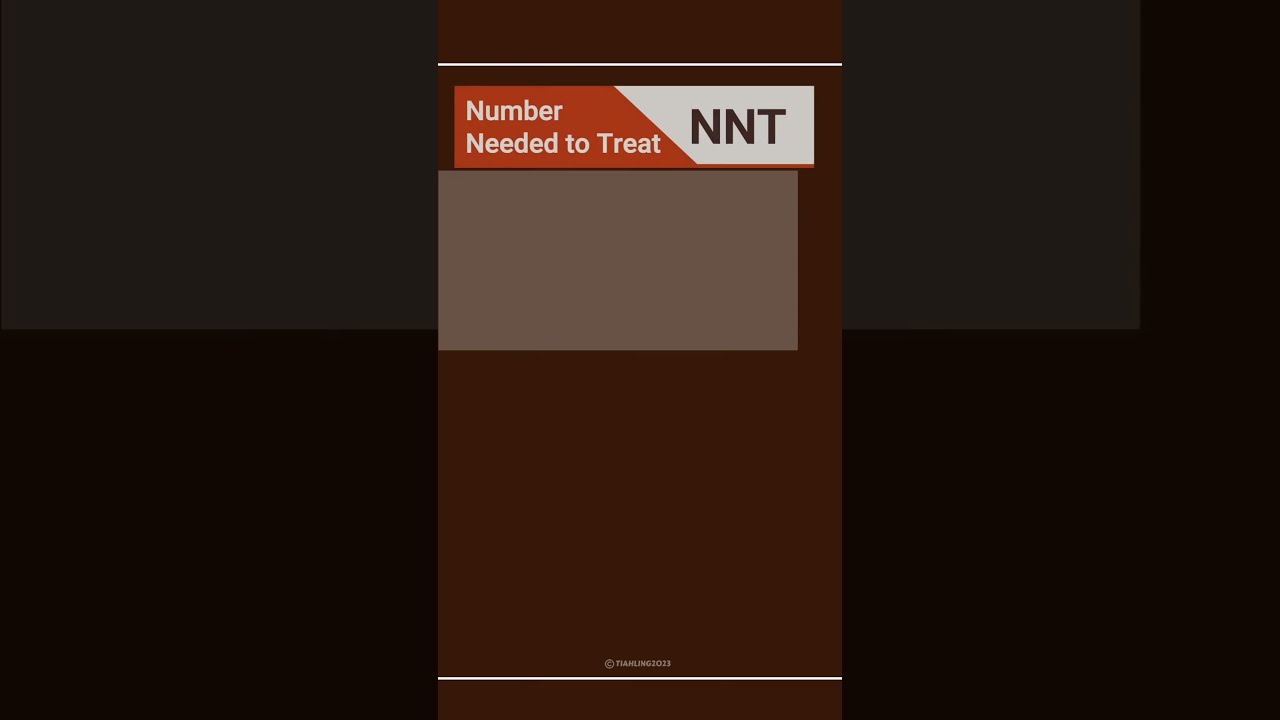The image depicts a detailed graphic organizer related to a clinical study. In the center, there is a brown rectangular box titled "Study Results." Below this, three pink boxes outline the outcomes: one labeled "Outcome," another "Tranexamic Acid (TXA), n=120," and a third as "Placebo, n=118." Beneath these, three white boxes detail the results for "Progressive Intracranial Hemorrhage (PIH)" with values "21 (17.5%)" and "32 (27.1%)." A larger white box underlines critical information, stating, "If we were to treat these 100 patients with TXA instead," accompanied by a visual with a mix of red, blue, and predominantly green dots. Annotations below illustrate the benefits, noting "Absolute Risk Reduction (ARR) = 9%" and highlighting a calculation: "Number Needed to Treat (NNT) = 11," showing "100/9 = 11." In the background, the left and right sides appear to magnify sections of the central box, emphasizing details such as the colored dots and the peripheral text.